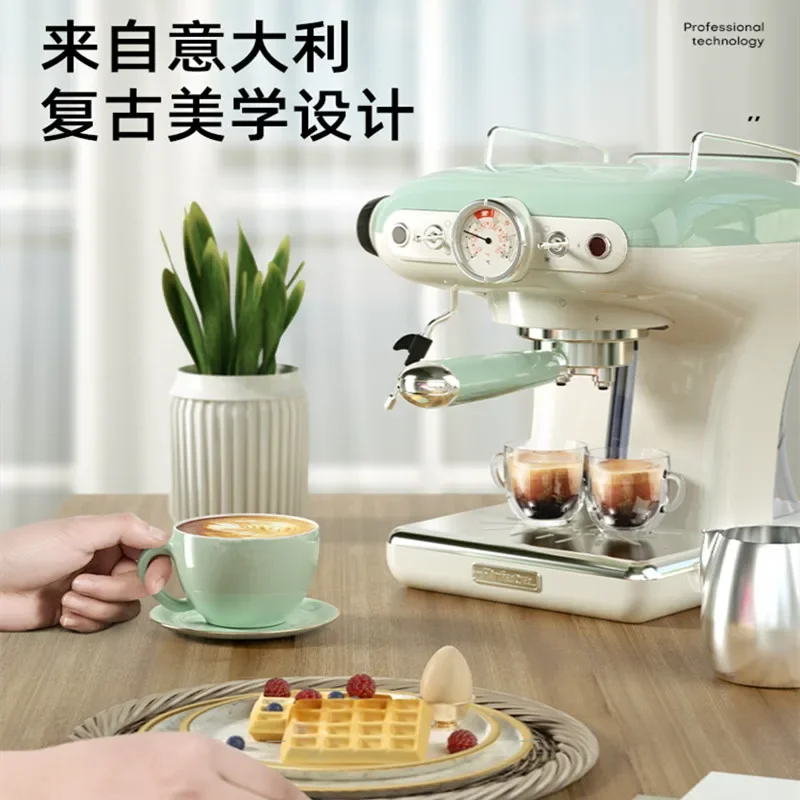This detailed photo captures a serene breakfast scene on a wooden counter. At the center, a retro-styled white espresso machine with light teal accents and stainless steel details stands proudly, epitomizing professional technology. The machine features two glass cups brimming with what looks like a rich espresso or latte. To the left of the espresso machine, framed by two rows of kanji characters, is a sliver pitcher likely containing cream for the coffee.

A woman’s hands appear prominently in the foreground. Her left hand holds a mint green cup with a matching saucer, filled with coffee boasting a latte art design, while her right hand steadies a plate. The plate is artfully arranged with a waffle topped with fresh raspberries and blueberries, and a boiled egg in an egg cup.

Adding a touch of nature, a small potted plant with spiky green leaves in a white pot is placed just behind the mug, enhancing the cozy ambiance. The background, subtly blurred, reveals a sheer-curtained window, adding to the overall modern yet warm aesthetic of the scene.